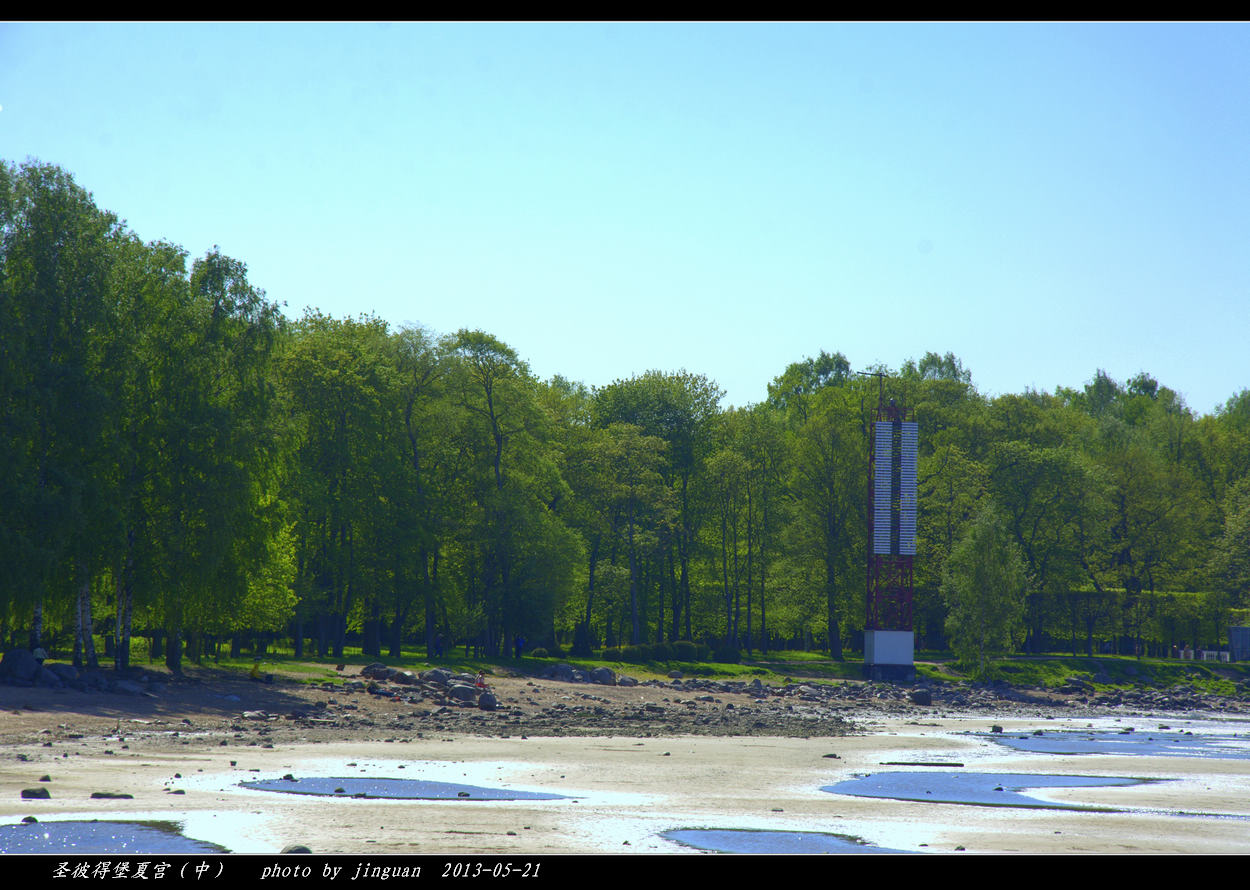The photograph depicts a serene coastal scene under a clear, blue sky devoid of clouds. In the background, a densely populated forest with vibrant green leaves extends across the horizon. The forest floor transitions into a rocky and sandy beach area marked by pools of water, suggesting the scene might be captured at low tide. The beach shows distinct areas where the tide normally reaches, evidenced by lighter and darker patches of sand and rocky dirt. A tall, multi-colored tower, possibly an observation or signal tower with a white cube base and striated panels, stands prominently near the right-hand side, partially obscured by the lush trees. Nearby, several cars are parked on the rocky ground, adding to the scene's detail. The far-right side of the image hints at some buildings partially hidden by the dense foliage, while some Japanese characters and the text "photo by Jingman 2013-05-21" are inscribed at the bottom of the photo.